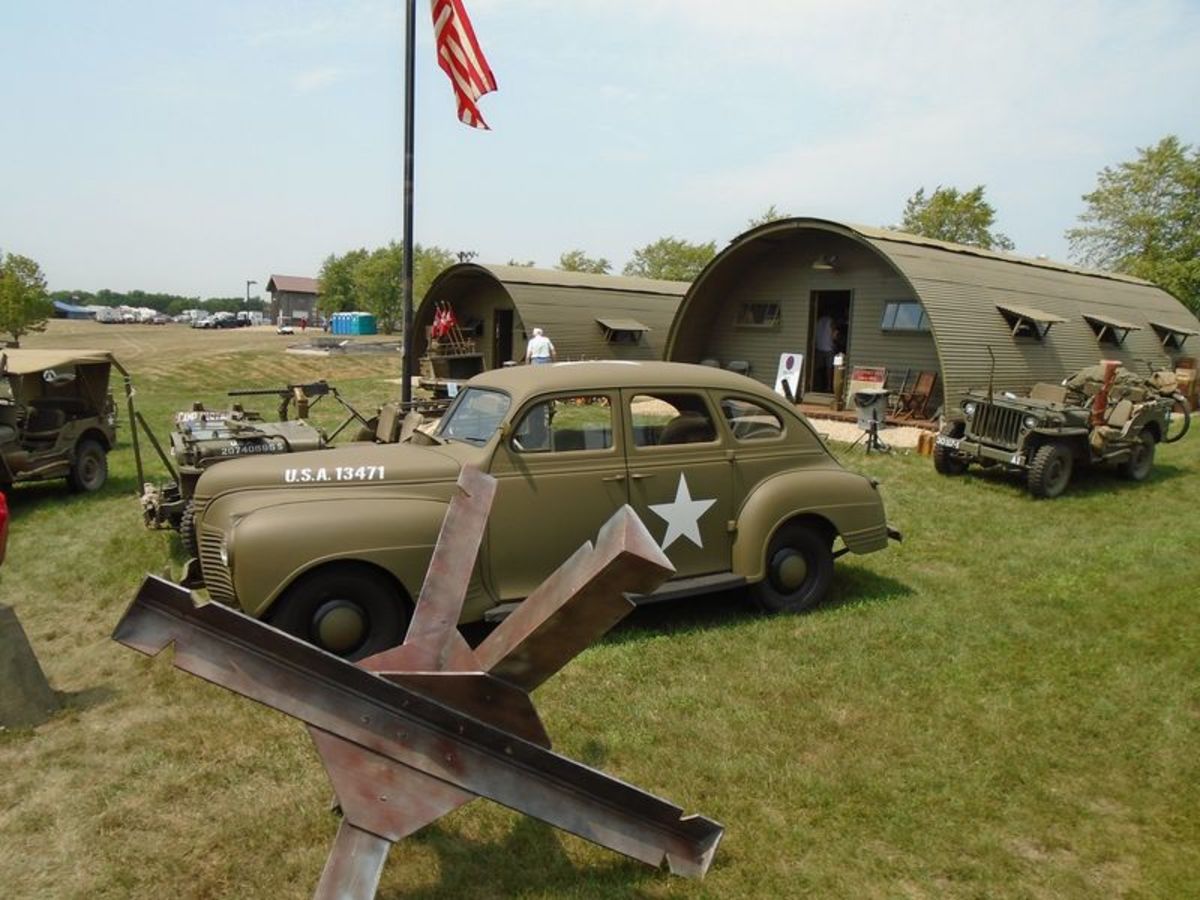The image depicts a World War II military museum scene set in a wide open field with lush green grass and trees in the background, suggesting it is summertime. In the foreground, a large, rusted metal object stands prominently, although its exact nature is unclear. Right behind it is a military-green, retro-looking car resembling an old Volkswagen or "punch buggy." The car's hood is marked with "USA 13471," and a prominent white star decorates the back left door. Surrounding the car are at least three other military vehicles, resembling old-school Jeeps and possibly a dune buggy, all painted in the same military green color. 

In the mid-ground, an American flag hangs from a pole, clearly visible. Two large, semi-circular military green buildings with central doors flanked by rectangular windows stand behind the vehicles. The doors of these structures are open, and a man in a white shirt is seen walking towards one of them. 

Beyond these buildings, there is a parking lot filled with modern cars and porta-potties, highlighting the historical nature of the scene. Overall, this photograph captures a detailed and evocative representation of military life and vehicles from a bygone era, set in a museum context.